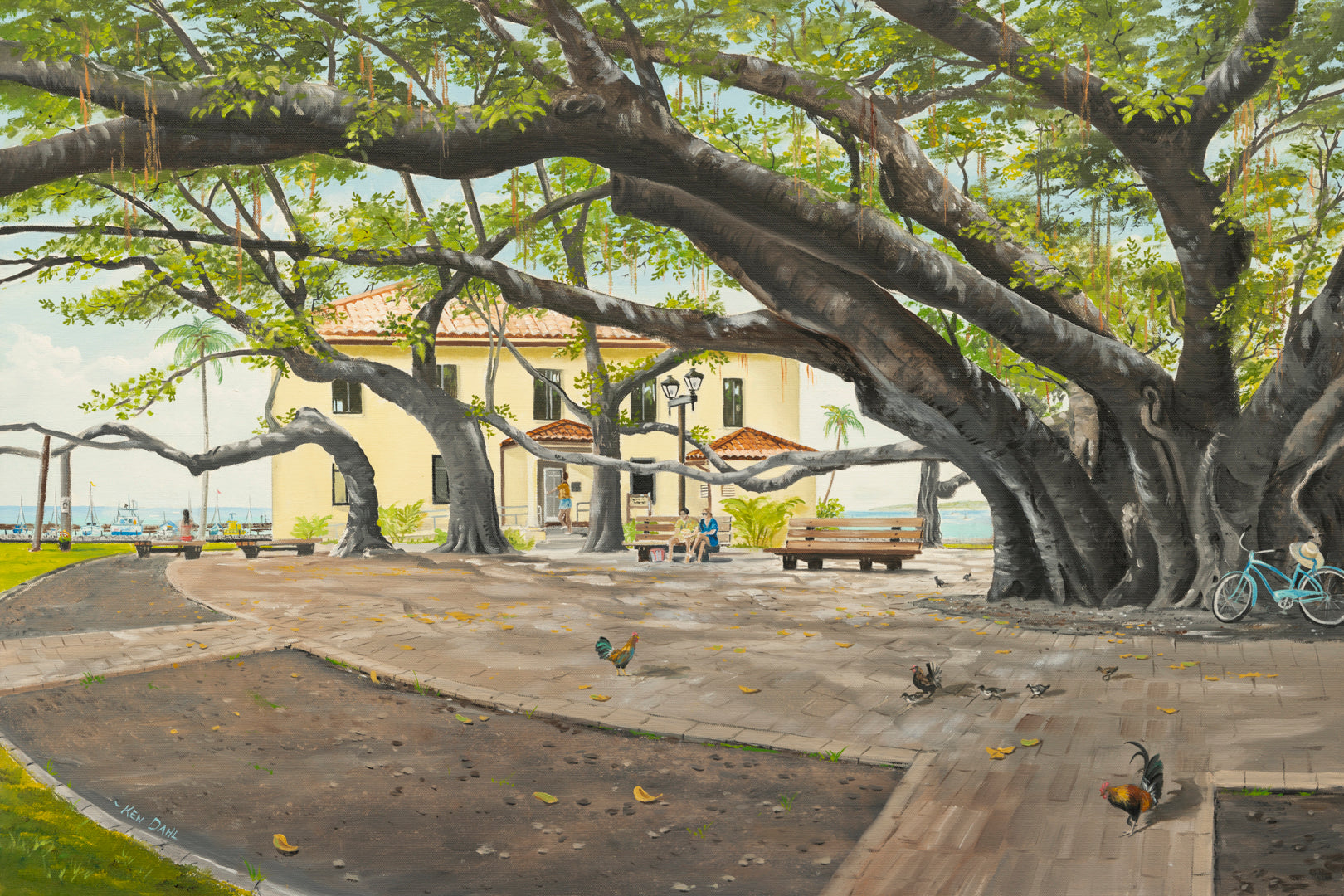In this vibrant, detailed artwork, an expansive tree with numerous sprawling branches dominates the scene, casting ample shade over a cobblestone pathway. Under the tree, a charming blue bicycle rests against its sturdy trunk, adorned with a summer hat featuring a blue ribbon perched on the bike seat. Along the pathway, several chickens, including two roosters, are energetically moving about.

Two wooden benches are situated beneath the tree's canopy; one is empty while the other is occupied by two women engaged in conversation. Near the benches, a tan-colored building with multiple windows stands, its yellowish hue complementing the sunny ambiance. This structure appears to be a small store or café, with another woman visible standing in the doorway. The backdrop extends to a serene body of water, possibly an ocean or lake, with a clear blue sky overhead. In the distance, a few small boats can be seen gently floating, and tall coconut palm trees sway by the water's edge, enhancing the serene, coastal atmosphere of this picturesque park-like setting.